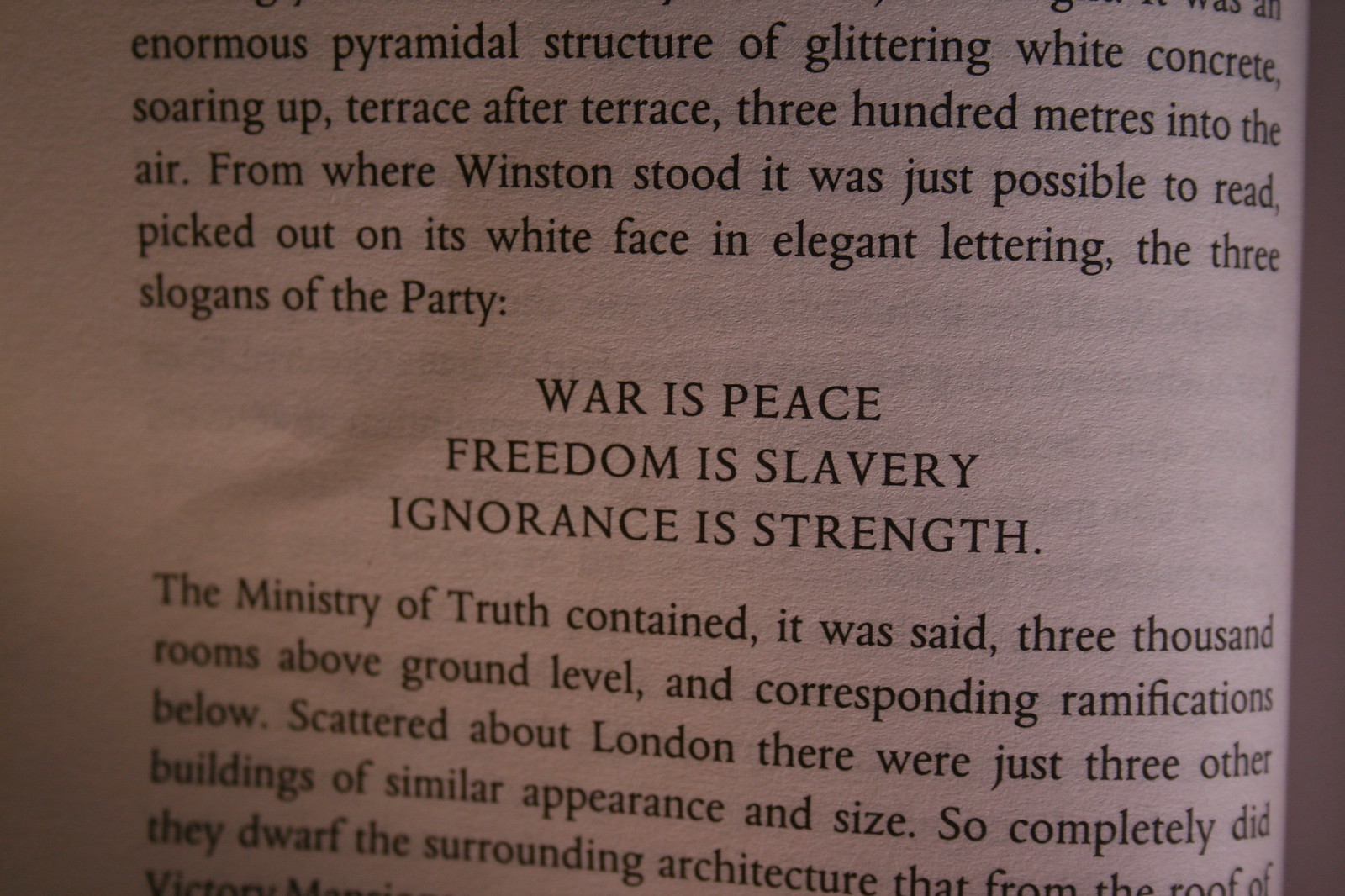This image depicts a rectangular section of a book page, taken at an angle where the inner seam of the book appears along the photo's right edge. The page itself, likely white, appears shaded gray or even brown due to the photograph's dark quality. The text within reads: "enormous pyramidal structure of glittering white concrete soaring up terrace after terrace, 300 meters into the air. From where Winston stood it was just possible to read, picked out on its white face in elegant lettering, the three slogans of the party—War is Peace, Freedom is Slavery, Ignorance is Strength." Below that, the passage continues: "The Ministry of Truth contained, it was said, 3,000 rooms above ground level and corresponding ramifications below. Scattered about London were just three other buildings of similar appearance and size. So completely did they dwarf the surrounding architecture that from the roof of..." The photo cuts off the remaining text. In this dimly lit image, black text stands out starkly against the shaded background, emphasizing the imposing description of the Ministry and its slogans.